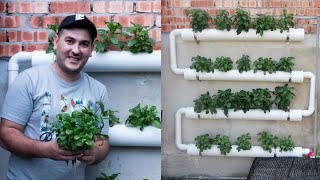The image features a rectangular split showing two photographs. On the left, there's a man smiling warmly, dressed in a gray short-sleeved shirt and a black baseball cap with an indistinct white emblem. He has short dark hair peeking out from under his cap. He's holding a small plant with green leaves in his hands, revealing his pale skin. The background is a red brick wall, partially covered with concrete, adorned with several white PVC pipes that form a serpentine shape. These pipes house numerous plants, suggesting a hydroponic setup. The right photograph offers a detailed view of this PVC pipe system, showing four main horizontal sections connected by smaller pipes via 45-degree bends. The upper tubes lead water into the lower sections, creating an efficient, sustainable gardening system. Various green plants flourish in the horizontal segments of the pipes, enhancing the innovative and visually appealing design against the mixed brick and concrete background.